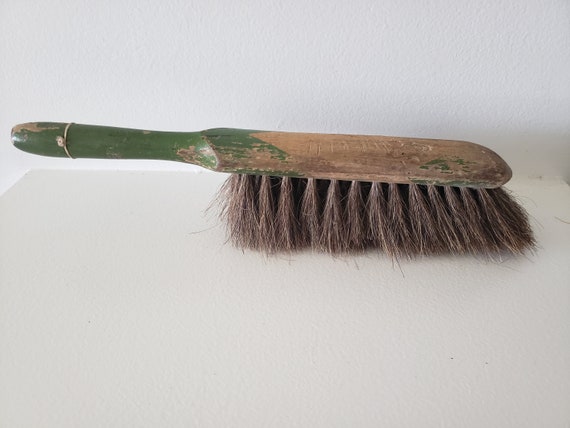The photograph captures an ancient wooden brush, possibly for hair or horse grooming, resting on a plain white surface against a white stucco wall. The brush features a heavily weathered wooden body with remnants of dark apple-green paint clinging to the handle, which tapers outward to its tip. The majority of the paint has eroded, revealing the natural brown wood beneath. The dense, large bristles are arranged in clusters, fixed to the underside of the wooden base, and appear bushed out like horsehair. A silver band encircles the base of the handle where it meets the bristles. The brush is positioned on its bristles, slightly elevating the handle off the surface, adding to the rustic and worn aesthetic depicted in this real-life photograph.